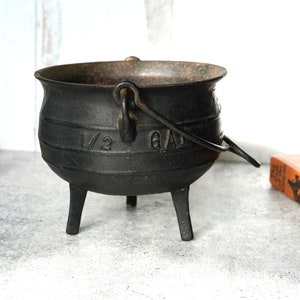This image features a black cast iron pot, closely resembling a traditional cauldron, complete with a sturdy handle cast into its side and three integrated legs for stability. Prominently embossed on the pot's side are the characters “1/2 GAL,” indicating its capacity. The pot sits on a smooth, possibly tiled surface, with an overall bright and sunny background. Beside the pot, a partial view of an orange book's spine is visible, adding a touch of color to the otherwise monochromatic setting. The photograph evokes an old-world charm, reminiscent of the kettle from the tale of the Three Little Pigs, standing alone in the simple yet bright scene.